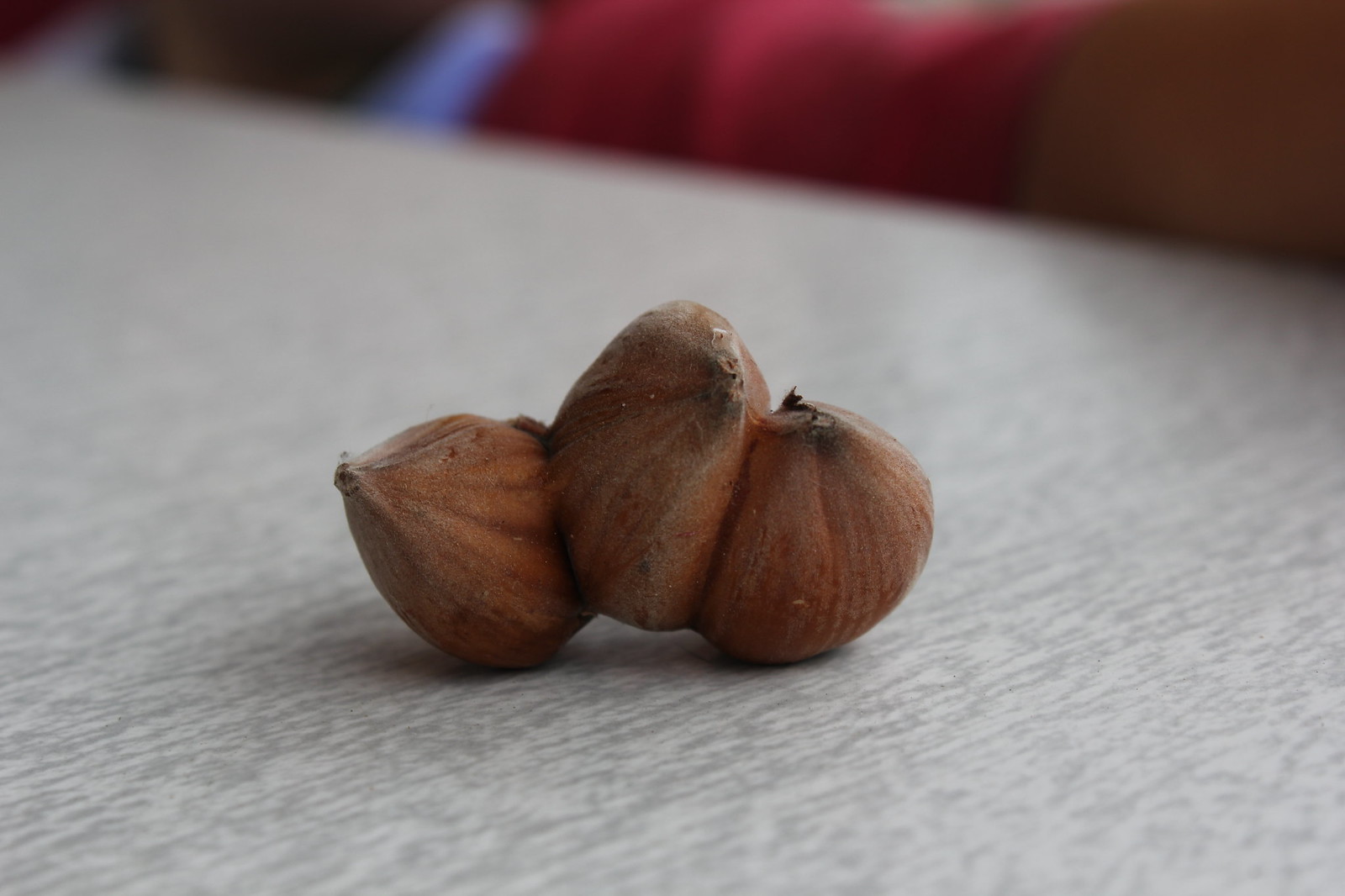This indoor close-up photo showcases a curious object on a white-gray, dappled countertop. The main subject appears to be a cluster of three light brown, slightly reddish-brown entities fused together, which could be interpreted as either dried garlic cloves, almonds, or figs. The central piece of this trio is elevated slightly higher than the other two pieces, which rest firmly on the tabletop. The focal point of the image is sharply defined, emphasizing the intricate texture and shape of these fused items, while the background fades into a soft blur of red and brown hues, adding depth to the composition.